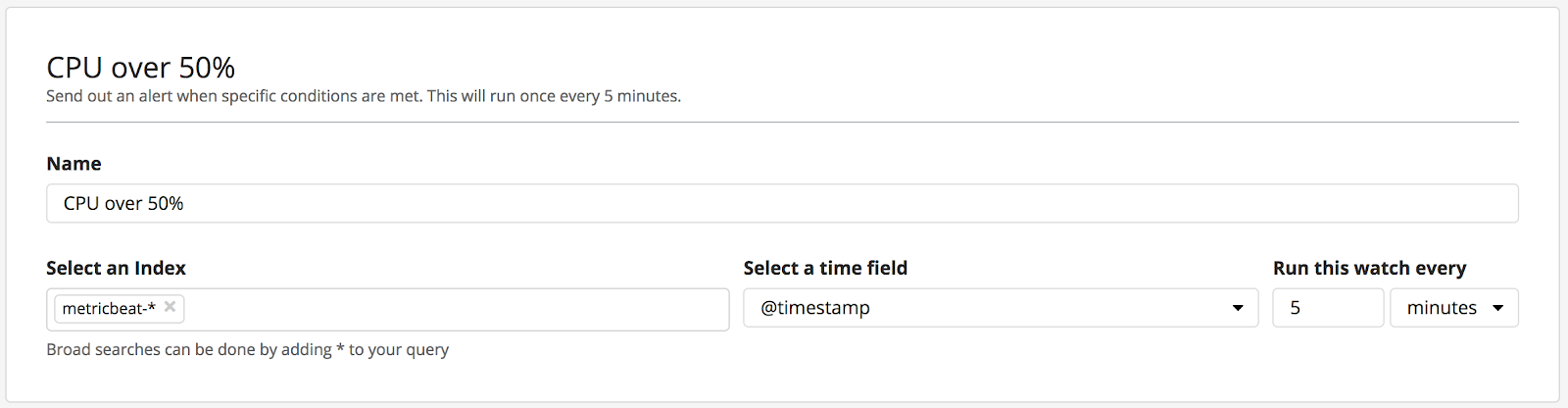Here is a cleaned-up, detailed caption for the image:

---

The image is a screenshot of a CPU notification alert interface, presented on a white background with a very thin gray border at the top and bottom edges. 

At the upper left of the notification, the largest text reads: "CPU over 50%." This heading is followed by the instruction: "Send out an alert when specific conditions are met. This will run once every five minutes." Beneath this, another thin gray line spans the width of the notification.

Further down, in bold text, the label "Name" appears, and just below this is the condition "CPU over 50%," again separated by a lighter colored line. Following this line, there are three bold columns: "Select an index," "Select a time field," and "Run this watch every."

Under the "Select an index" column, the option "metricbeat" is selected, marked with a star and an 'X' for closing this option. The "Select a time field" column instructs to "Add timestamp." The "Run this watch every" column features a down arrow option, with "5" selected from a drop-down menu and the time unit set to "minutes," also selected from another drop-down menu.

At the bottom, an additional guideline reads: "Broad searches can be done by adding a star to your query."

The screenshot showcases a very wide field, with no other elements visible on the page.